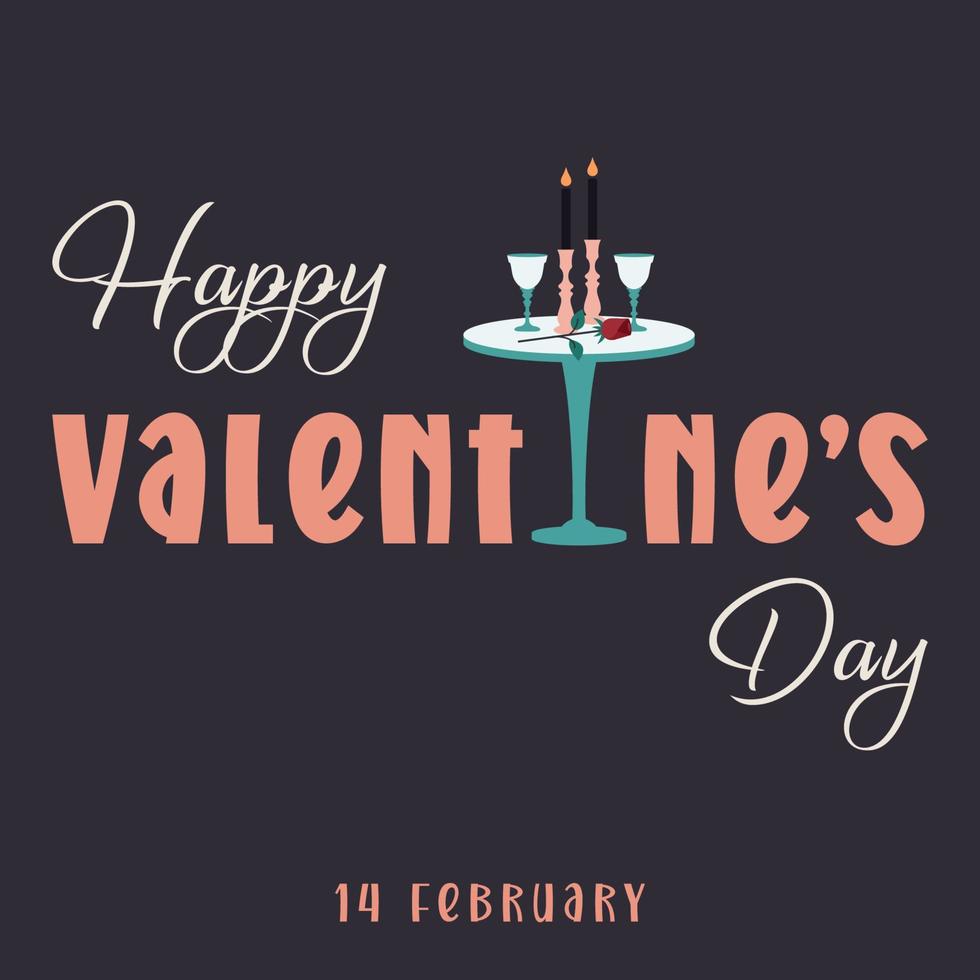This cartoon illustration celebrating Valentine's Day features text arranged artfully across a predominantly black background. At the top left, "Happy" is written in elegant off-white cursive. The word "Valentine's" spans the center in a playful pink font, with the "I" ingeniously represented by the single leg of a small, simplistic green table. Atop the table, which has a blue or white rounded top, rests a romantic setup: two black pillar candles in pink holders, two wine glasses, and a long-stemmed red rose. Just below "Valentine's," to the right, "Day" is inscribed in matching off-white cursive. At the very bottom, centered, the date "14th of February" is displayed in the same pink hue as "Valentine's." The composition creates a whimsical yet cozy Valentine's Day greeting.